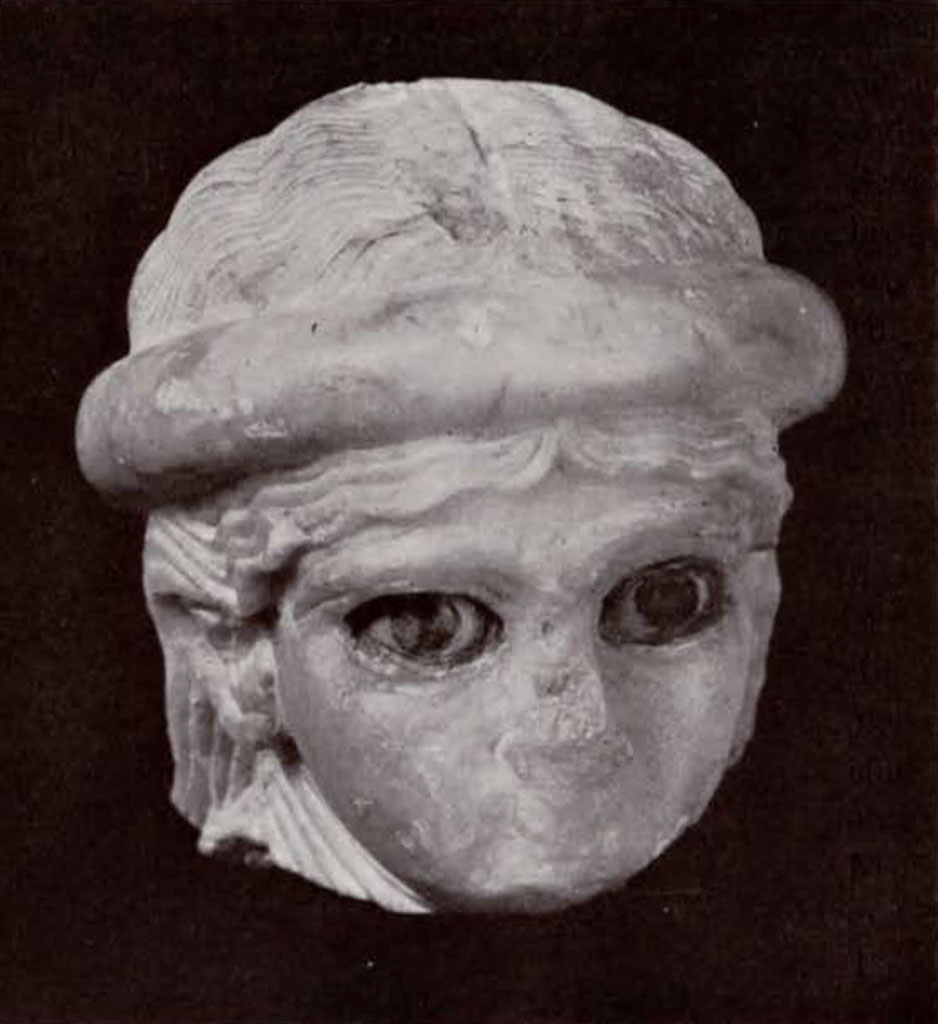This close-up photograph showcases the head of a sculpture set against a stark black background, emphasizing the intricate details of the artwork. The head, appearing to be carved from a grayish-white material such as marble or cement, embodies characteristics reminiscent of ancient Greek or Roman art. The figure, possibly representing a child or young woman, is adorned with a headband that encircles long, curly hair, artistically rendered in delicate, wavy lines. The eyes are strikingly large, with dark pupils that draw immediate attention. Notably, the nose of the sculpture is damaged, with the tip chipped off, and there is no defined mouth, as if never carved or eroded over time. This lack of a mouth combined with the childlike, juvenile facial features adds a haunting, enigmatic quality to the artwork.